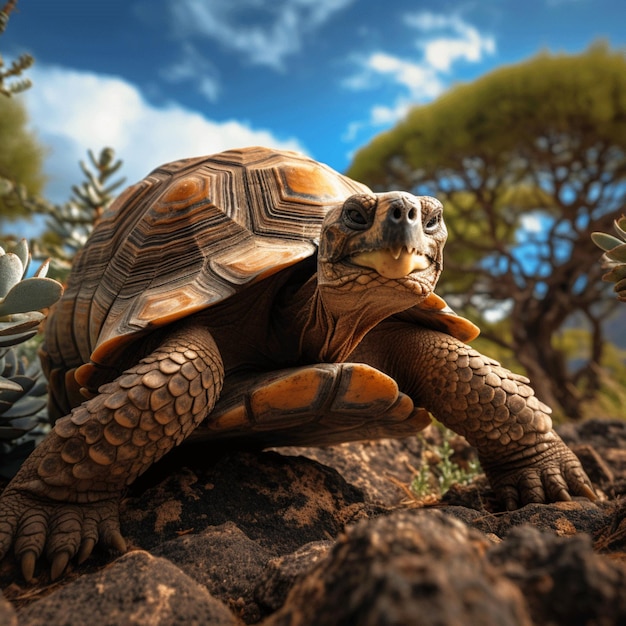This highly detailed, close-up, realistic photograph of a tortoise captures the creature outdoors during the day. The tortoise, with its scaly, brownish-orange legs extended in front, walks purposefully across a textured soil foreground peppered with dark and lighter brown rocks, resembling charcoal. Its head, characterized by a beak-like face with black eyes and a dark nose, emerges confidently from its textured shell, which features a mesmerizing geometric pattern of rectangles and near hexagonal shapes, in hues of golden orange, yellow, and darker browns. The shell’s underside displays contrasting yellow and black tones. The tortoise’s gaze meets the camera directly, revealing wrinkles on its neck and what appears to be an open mouth with a hint of a tan tongue. The serene background includes a clear blue sky adorned with white clouds, flanked by trees in the top corners and various succulent plants on the left, providing a tranquil, natural backdrop to this lifelike capture.